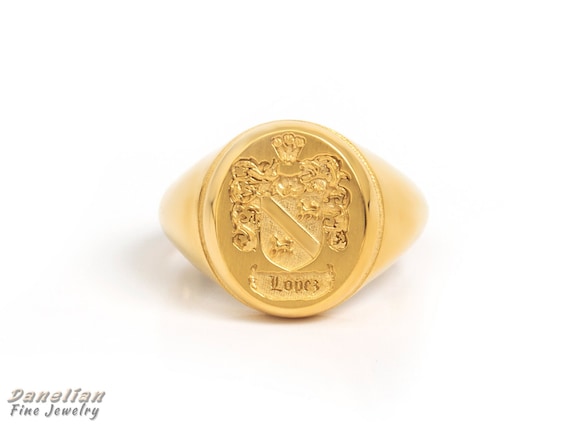This detailed image depicts a gold signet ring prominently displayed in an advertisement for Denelian Fine Jewelry, as indicated by the small silver logo located in the lower left-hand corner of the photograph. The ring features a round center with tapered sides and is entirely gold. The centerpiece of the ring showcases an ornate coat of arms, which includes a detailed shield flanked by intricate decorative elements and topped with a three-pronged crown. Underneath the coat of arms, the name "Lopez," spelled L-O-P-E-Z, is elegantly engraved in a calligraphy-type font.